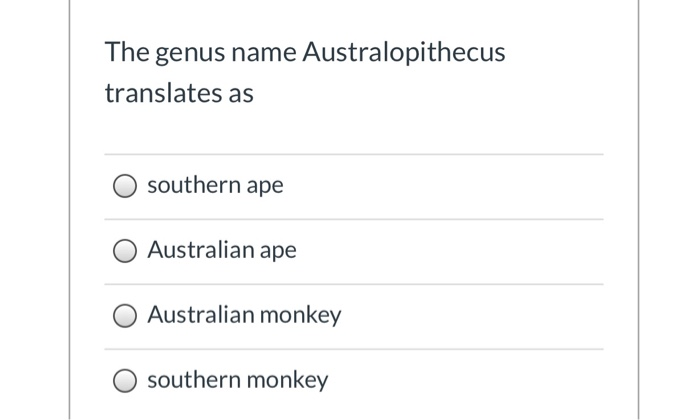The screenshot captures a small section of a website with a white background and very light gray vertical lines on both the left and right sides, indicating that this is just a portion of a larger webpage. The headline, positioned in the left margin, is in dark gray and reads "GENUS name." The genus name, "Australopithecus," is presented in all caps, and though the spelling is clarified (A-U-S-T-R-A-L-O-P-I-T-H-E-C-U-S), pronunciation guidance is not provided.

Below this headline, a light gray horizontal line extends from left to right. Underneath the line, there is a gray dot followed by the phrase "Southern Ape." This pattern repeats in the same format: a light gray line, a gray dot, and the terms "Australian Ape," "Australian Monkey," and "Southern Monkey," listed vertically one below the other on the left side of the screen.